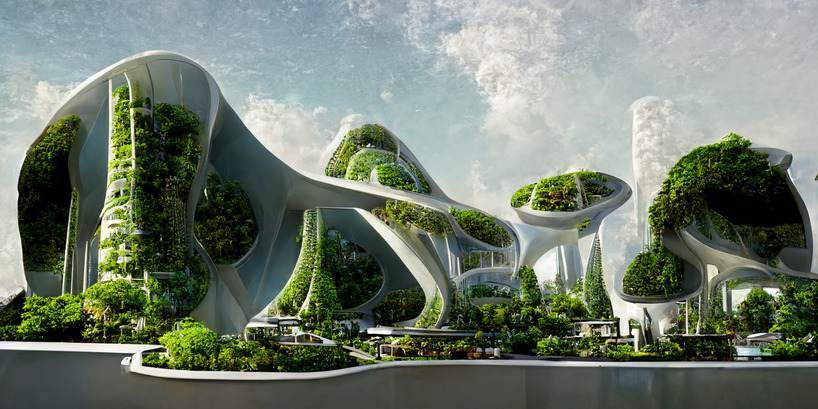The image depicts a futuristic cityscape featuring an array of large, white, curvy structures that evoke a sense of advanced architecture akin to scenes from "The Jetsons." The buildings are nestled within and adorned by abundant greenery, with trees, bushes, and vines seamlessly integrated into the design. These organic elements intertwine with the sleek, modern forms, creating a biomechanical aesthetic where nature and artificial constructs harmoniously coexist. The structures are built atop a high, curvy white wall and extend upward, some forming circular shapes reminiscent of floating islands. The sky above is a serene light blue, dotted with fluffy white clouds, enhancing the ethereal quality of the scene. The combined effect is that of a visionary, eco-friendly urban environment, possibly AI-generated, illustrating a beautiful and sustainable future.